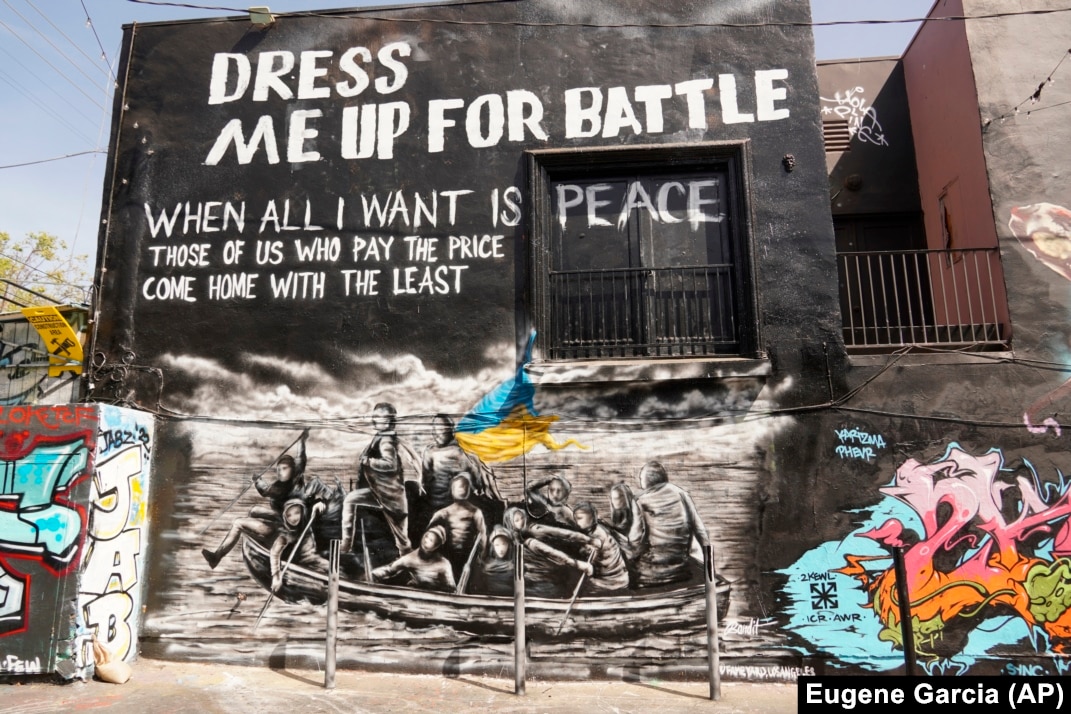In this image, we see the side of a building adorned with a striking mural. The focal point of the artwork is a section painted black with white text that reads, "Dress me up for battle, when all I want is peace. Those of us who pay the price come home with the least." The word "peace" is prominently displayed over a double doorway, which is enclosed by a small balcony. Below this textual element, there is a vivid painting of civilians paddling a boat on a body of water, featuring a flag that is yellow and blue. The scene is set against a background of additional graffiti art on both sides. The mural is signed "Eugene Garcia (AP)" in the bottom right corner. A concrete sidewalk, in a white-tan hue, runs alongside the base of the building. Sparse glimpses of the sky are visible in the upper corners of the image.